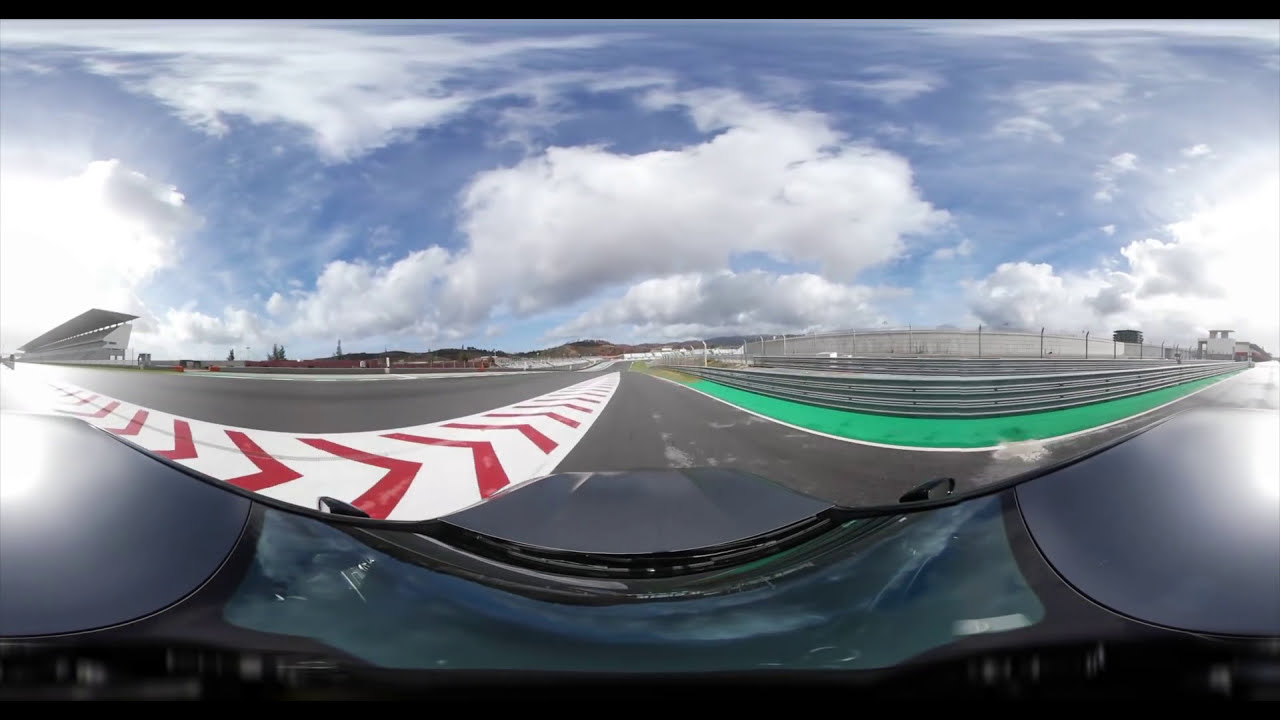The image is a detailed view from the point of view of someone driving a race car on a racetrack, potentially resembling the Indianapolis road course. The bottom fourth of the photograph showcases the front dashboard and hood of a black and blue car. Directly ahead lies a gray road, flanked on the left by a white barrier featuring red arrows and a gray guardrail with green accents. In the distance, to the left, there are grandstands or bleachers, hinting at a larger stadium environment. On the right side, a guardrail extends until it disappears out of the frame, accompanied by red rumble strips in the distance. The sky occupies the top half of the image, painted light blue with scattered white clouds. The photograph, six inches wide and four inches tall, is framed by a thin black border at the top and shows signs of being a composite image, as if viewed from two different angles stitched together. The scene is devoid of any attendees, suggesting a practice or preparation session on the racetrack.